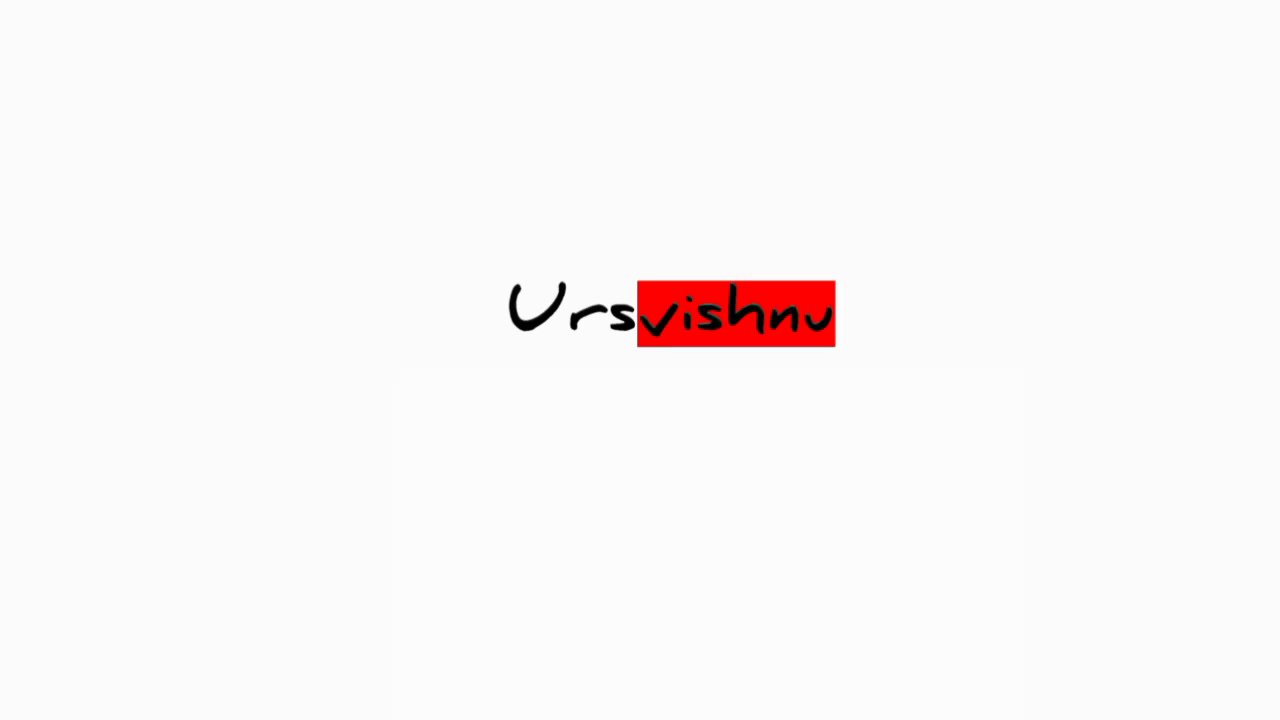The image features a single word, "URS-VISHNU," in handwritten black text, with the letters "URS" capitalized. The word is situated in the middle of a large horizontal rectangle shaded in light gray. The "VISHNU" portion is distinctly highlighted within a red rectangular box, creating a noticeable contrast against the light gray background. The letters are not cursive but retain a handwritten style, giving a unique and stylized appearance to the text. The rest of the image retains the light gray background with no additional text or elements.